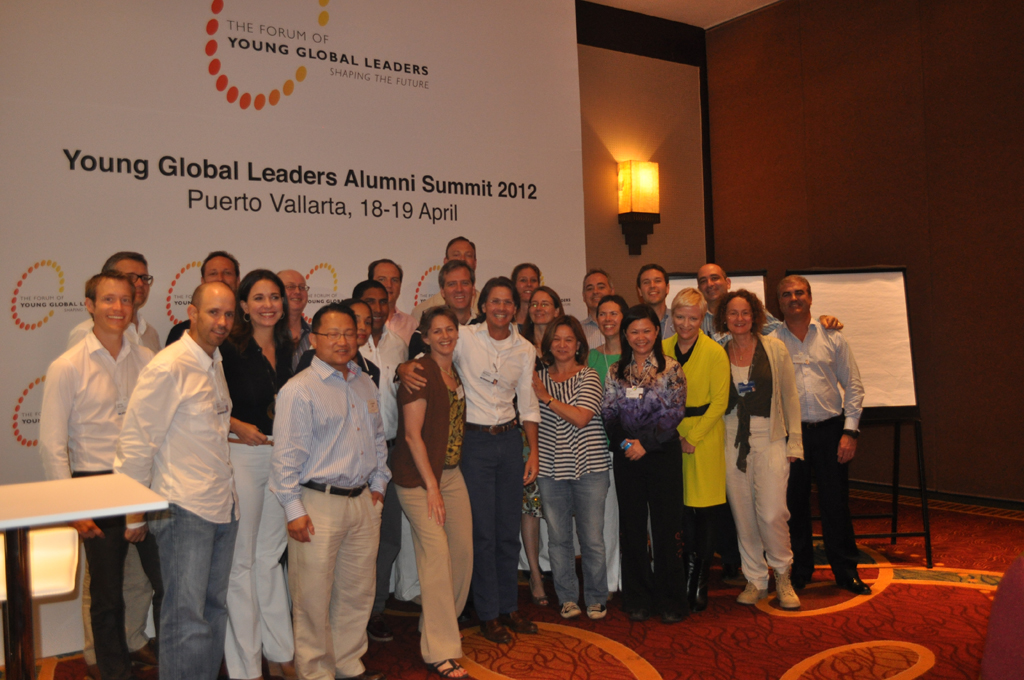The image depicts a horizontally aligned group photo taken at the Young Global Leaders Alumni Summit 2012, held in Puerto Vallarta on April 18-19. Approximately 20-30 young attendees, a mix of men and women, are standing in a hotel reception area in front of a large white banner. The banner prominently features the event’s title in bold black letters: "Young Global Leaders Alumni Summit 2012," with the phrase "Forum of Young Global Leaders, Shaping the Future" written above it. The lower portion of the banner, featuring various circular logos, is partially obscured by the group. The backdrop features a two-toned wall—brown on the right side and beige on the left—with a reddish carpet covering the floor. A notable detail is a wall lamp casting a yellow light from a cubicle-shaped glass cover. The group appears mostly formally dressed, with the exception of one woman in the front wearing jeans and a striped T-shirt. A white table is visible on the lower left, and a stand holding large paper is on the right side of the image. Some attendees have their arms around each other, showcasing a sense of camaraderie.